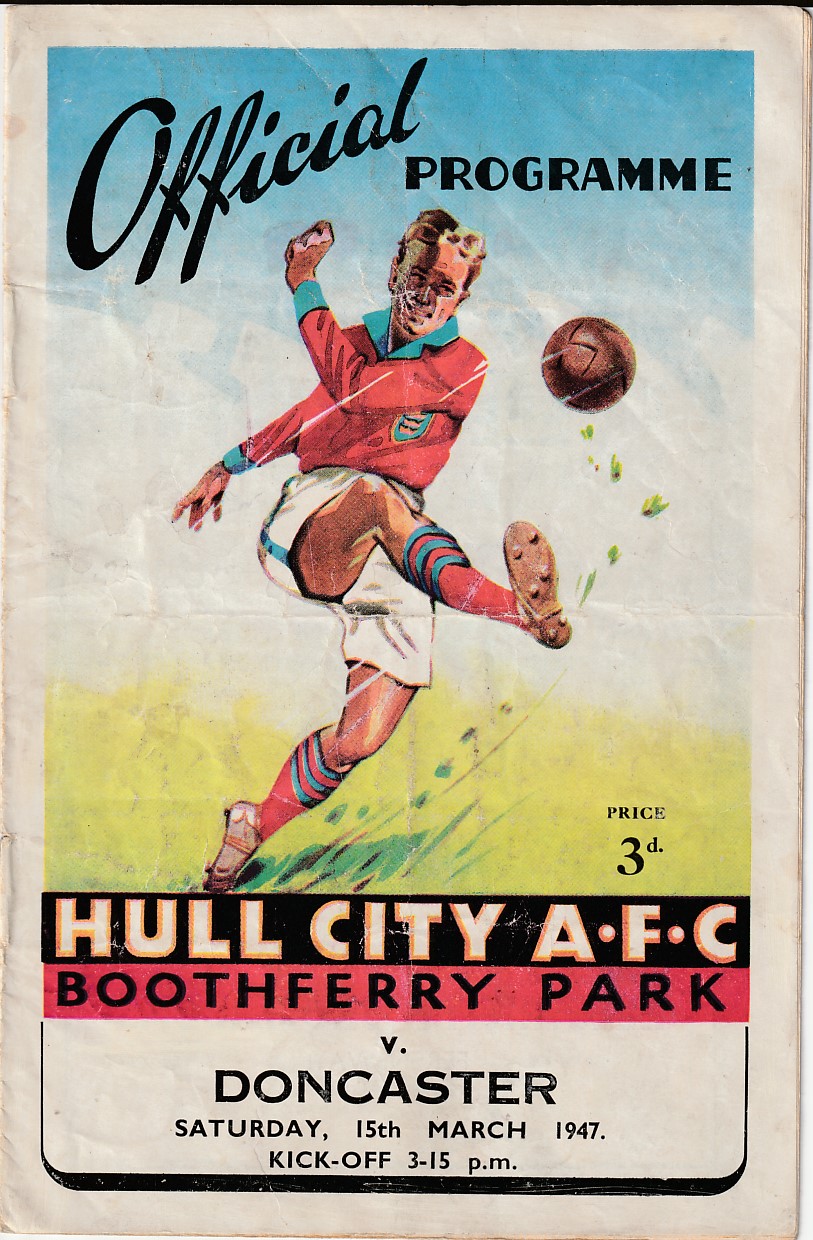This image depicts an official soccer match program with a detailed artistic drawing of a soccer player. The top portion is blue with black lettering that reads "Official Program." Below this heading is a dynamic illustration of a player in mid-kick, wearing a long-sleeved red jersey with a white stripe and a blue collar. His white shorts feature a blue stripe, and he sports red socks with blue stripes. The player’s right leg is extended upward, as if he's about to make contact with a brown, bronze-colored soccer ball suspended in the air. His left leg is firmly planted on the ground. The background transitions from blue at the top to white in the middle and yellow at the bottom, giving the image depth and contrast. Beneath the illustration, against a black backdrop with white print, it says "Hull City AFC." Below this, on a red background with black text, it reads "Booth Ferry Park vs. Doncaster." Further down, written in black text on a white background, are the details: "Saturday, 15th March, 1947, Kickoff 3.15 PM." In the bottom right corner, it states "Price 3D." The overall design captures the essence of mid-20th-century sports artistry and event promotion.